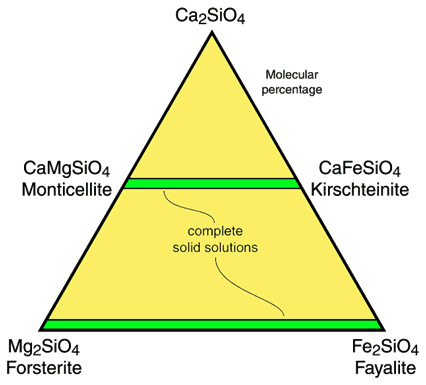This image features a large, equilateral triangle with multiple labeled sections and a complex color scheme. The central part of the triangle is predominantly yellow, intersected by two distinct green stripes; one stripe runs horizontally across the middle, and the other is located at the triangle's base. Additionally, a small, blue squiggly line traverses the triangle, drawing attention to the text "complete solid solutions" within the yellow area. At the apex of the triangle, in bold black font, the chemical formula "Ca₂SiO₄" is prominently displayed. The triangle's sides are annotated with molecular percentages: "CaMgSiO₄" labeled as Monticellite, "CaFeSiO₄" referred to as Kerstenite, "Mg₂SiO₄" denoted as Forsterite, and "Fe₂SiO₄" indicated as Fayalite. These form a comprehensive mineralogical map, detailing the solid solution phases within the system presented.